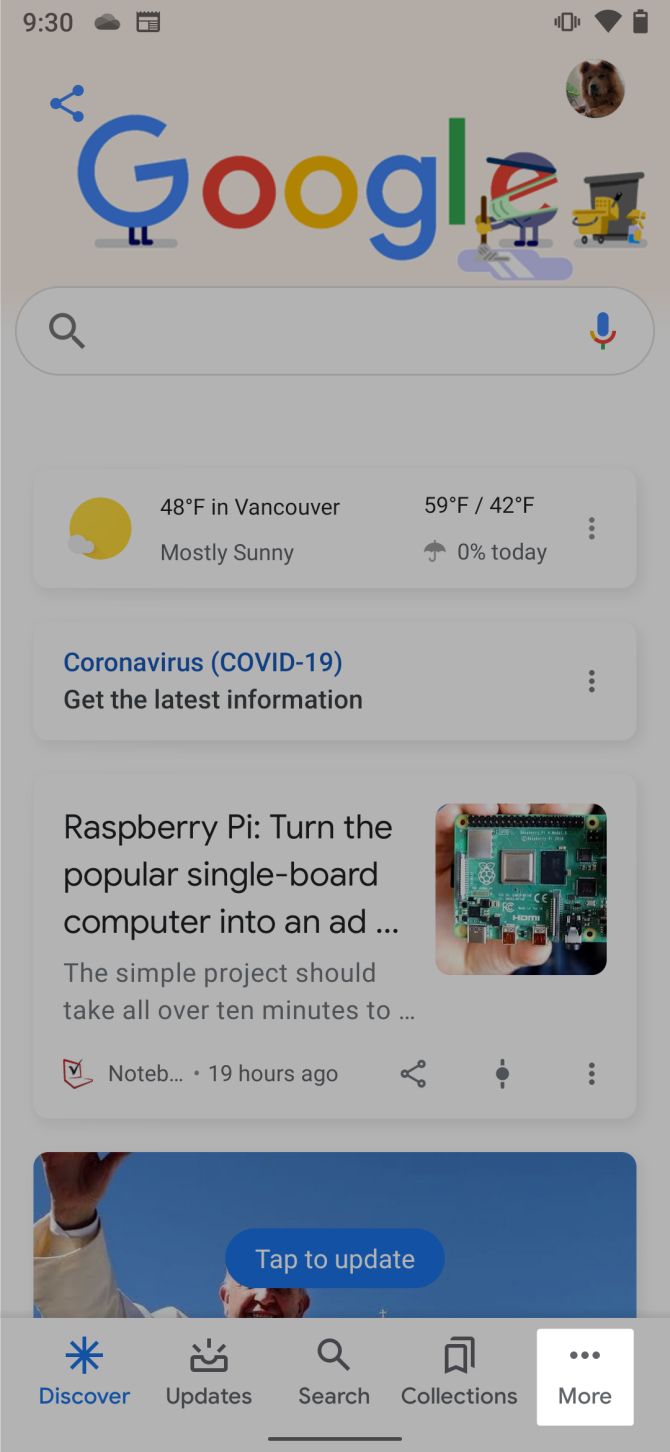At the top of the screen, there is the Google logo with the letters in the following colors: the first 'G' is blue, the first 'O' is red, the second 'O' is yellow, the second 'G' is blue, the 'L' is green, and the 'E' has segments of red, blue, and green, with additional blue at the bottom resembling pants. In the top right corner, there is a profile picture of a dog, followed by icons for vibration mode, full WiFi signal, and an almost fully charged battery with a small portion unfilled. 

On the top left, the time displays as 9:30, next to icons for a cloud and a rectangle. Below the Google logo, there is a search bar featuring a microphone icon and a magnifying glass icon. 

Beneath the search bar, it shows the temperature as 48°F in Vancouver, with a high of 59°F and a low of 42°F, along with a 0% chance of precipitation, indicated by an umbrella icon. The weather description reads "mostly sunny." 

Following this, there is a brief news update on Coronavirus (COVID-19), urging users to get the latest information. Another article headline mentions "Raspberry Pi turns the popular single board computer into an ad," describing a simple project estimated to take over 10 minutes to complete.

Lastly, the screen displays four highlighted options with three dots next to them: 'Collections,' 'Search,' 'Updates,' and 'Discover.'